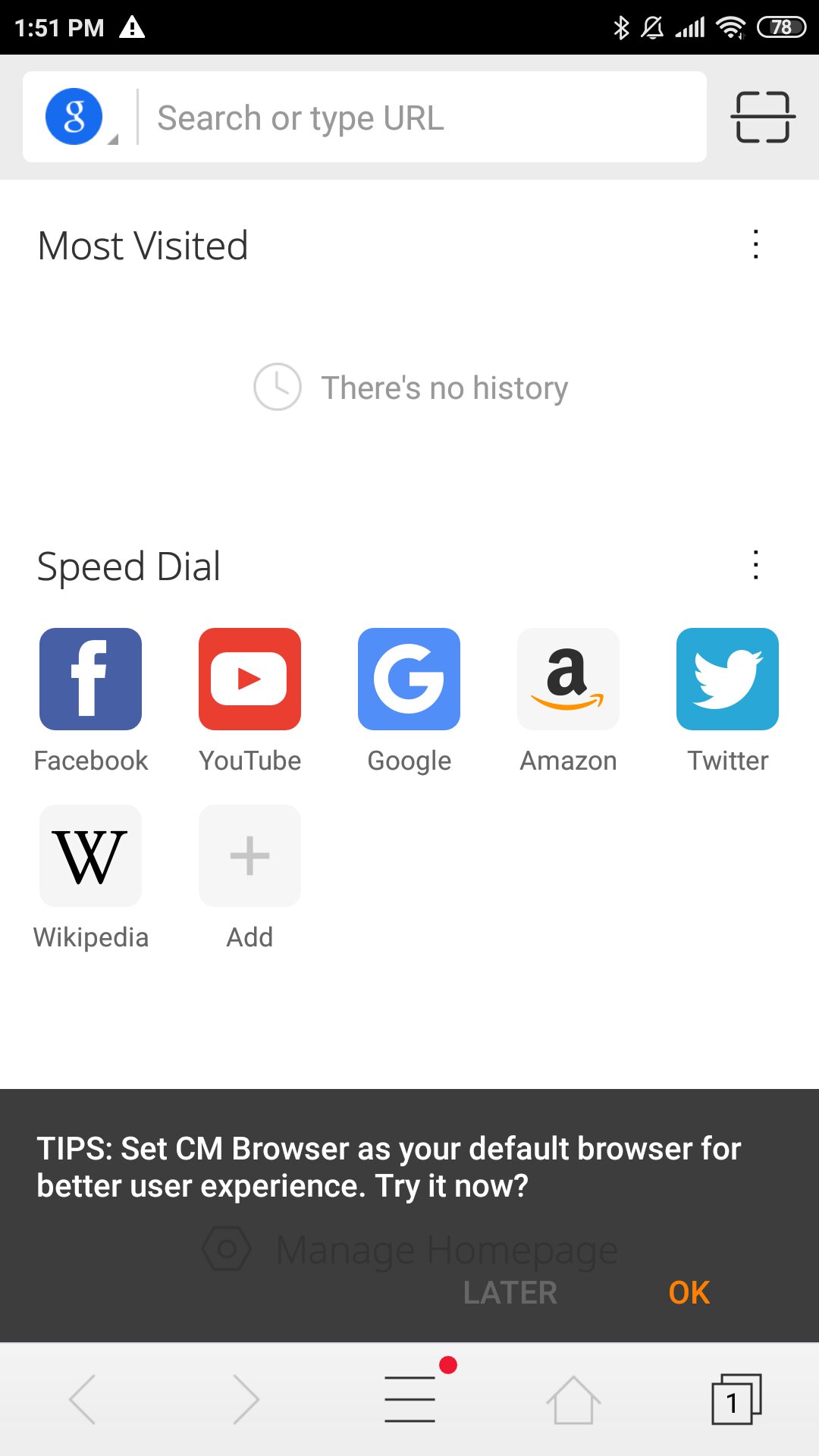The image depicts a screenshot of a smartphone internet browser interface. At the top, there is a Google search bar. Below it lies a "Most Visited" section, which currently indicates "No History." Further down, there's a "Speed Dial" section featuring various icons for frequently accessed websites, including Facebook, YouTube, Google, Amazon, Twitter, and Wikipedia. An ad icon is also present in this area.

At the bottom part of the image, a popup titled "Tips" prompts the user to set "CM Browser" as the default browser for an enhanced user experience, offering two action buttons: "Later" on the left and "OK" on the right. In the background behind the popup, text reads "Manage Home Page."

The bottom of the screen houses a navigation bar with several buttons. From left to right, these are: a left-facing arrow for backwards navigation, a right-facing arrow for forward navigation, a three-line button often used for accessing additional options or a menu, a home button to return to the homepage, and a tabs button represented by a square overlapping another square with the number "1" indicating the current number of open tabs.